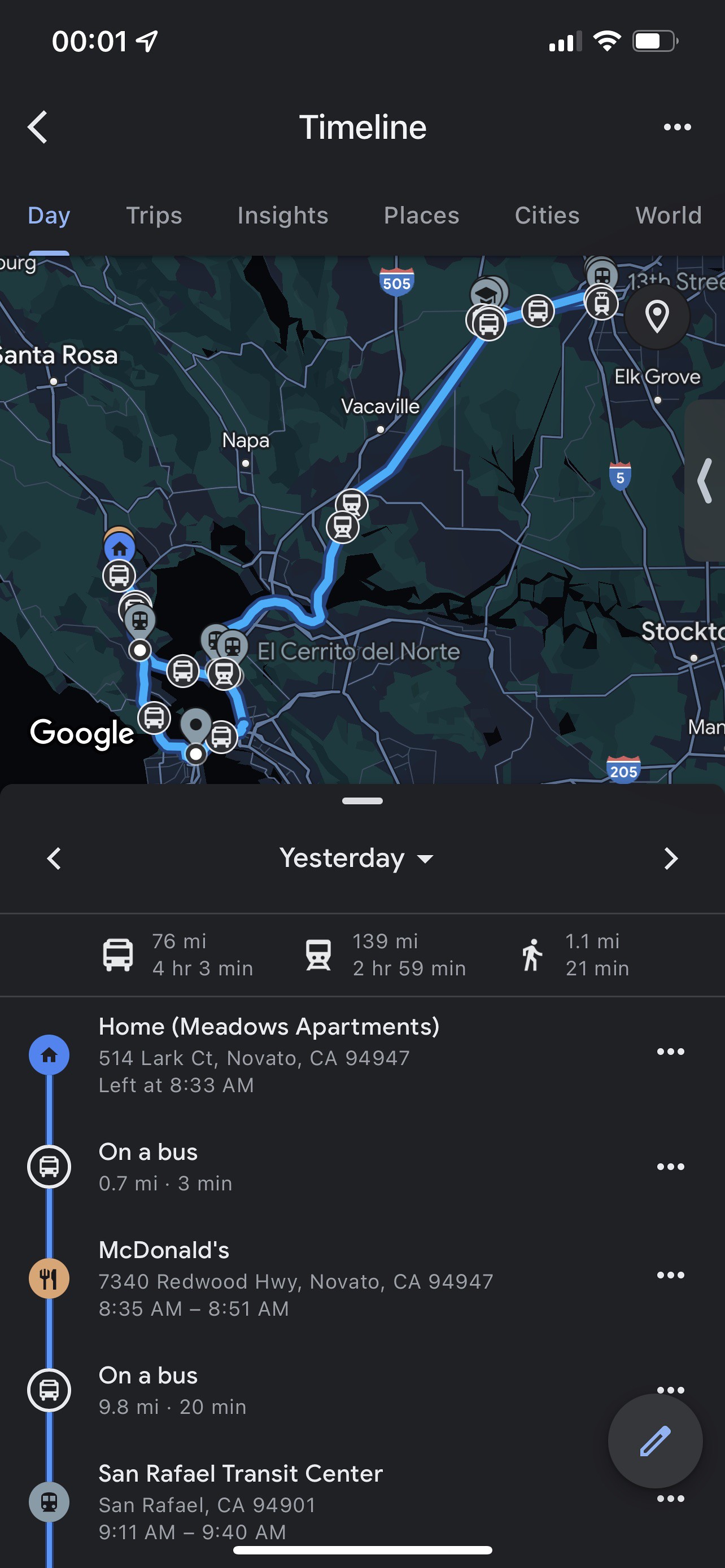The screenshot captures a detailed map of a journey from Novato, California to Elk Grove. The top portion of the image displays a Google Map in dark mode. The map is predominantly black with green areas indicating vegetation, contrasting sharply with the light blue trail that marks the route. Along this route, various stops and icons are visible. Place names like Santa Rosa, Napa, Vacaville, Elk Grove, and Stockton appear in white text.

Below the map, a section titled "Yesterday" features navigation arrows pointing left, right, and down. This section provides a summary of the trip's segments: 76 miles by bus in four hours and three minutes, 139 miles by train in two hours and 59 minutes, and 1.1 miles on foot in 21 minutes. 

Further down, details of five specific stops are listed: departure from home, boarding a bus, visiting McDonald's, taking another bus, and arriving at the San Rafael Transit Center.